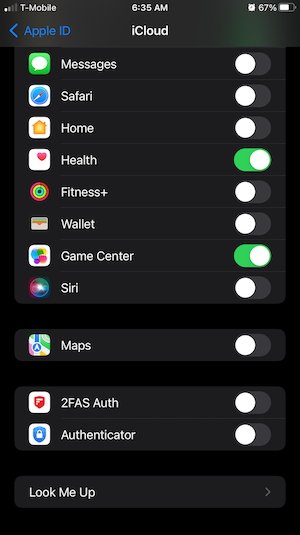This is a detailed screenshot of an iPhone screen displaying the iCloud preferences window. The image has a black background and is oriented vertically. 

In the upper left-hand corner, the signal strength icon shows one bar and a slightly filled second bar, with T-Mobile listed as the carrier. At the top center, the time is displayed as 6:35 a.m. In the upper right-hand corner, there's an alarm clock icon followed by a battery indicator displaying 67% charge.

The iCloud preferences window dominantly showcases a blue header with an Apple ID and a back caret arrow pointing left. "iCloud" is prominently written in white text below this. Underneath, a list of apps is shown with their respective iCloud backup statuses. The apps listed are Messages, Safari, Home, Health, Fitness Plus, Wallet, Game Center, Siri, Maps, 2FASAUTH Authorization, and Authenticator.

Each app name is accompanied by a radio slider button indicating whether the app data is being backed up to iCloud. All the sliders are in the "off" position, with white circles on the left side of the ovals, except for Health and Game Center. These two apps have their sliders moved to the right, indicating they are currently being backed up to iCloud, evidenced by the green background inside their respective ovals.

Overall, the screenshot provides a clear view of the iCloud backup settings on an unspecified model of an iPhone, showcasing which apps are included in the iCloud backups.